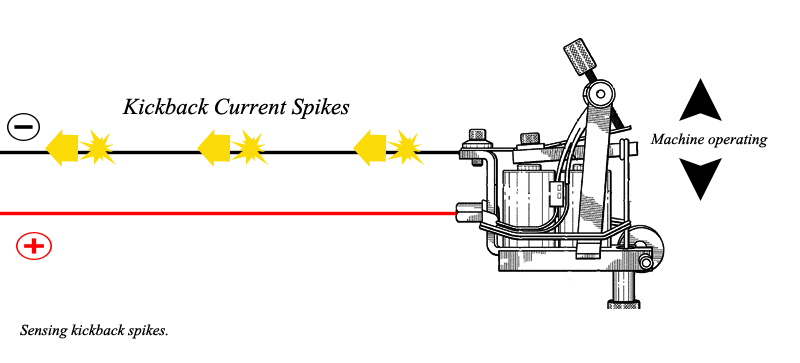The image is a detailed technical diagram, illustrating the movement of belts, wheels, pulleys, and cables within a mechanical engine. Two horizontal lines, identified as cables, emerge from the contraption, extending to the left. The top line is black and labeled as negative; it features three clusters of yellow arrows and starburst symbols along its length, indicating kickback current spikes. The bottom line is red, labeled as positive, and remains unmarked. The machine, reminiscent of a telescope with spinning parts, displays various components and their interactions, including arrows pointing upwards and downwards labeled "machine operating" in black. The entire setup is shown without any background, emphasizing the components and their connections.